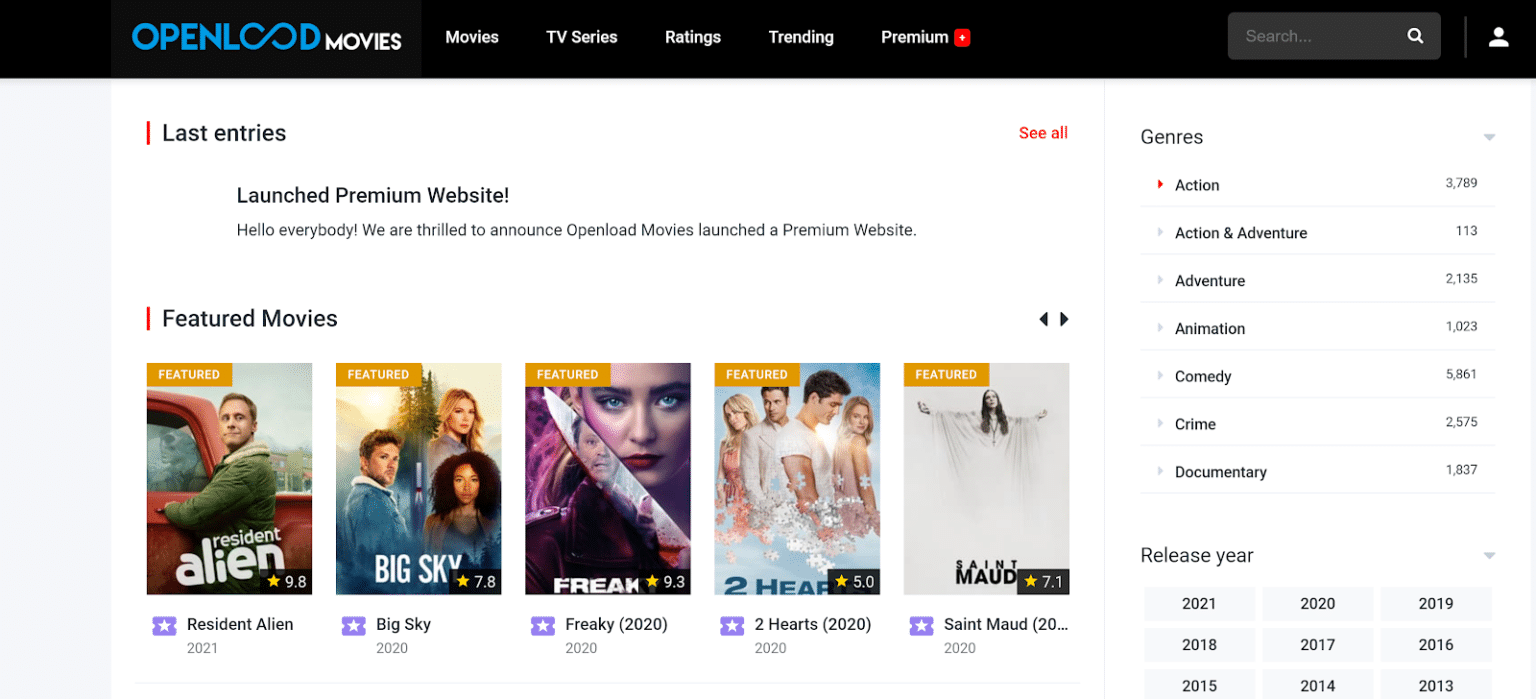This image depicts the homepage of a movie website featuring a sleek design with a white background and a prominent black border at the top, serving as the menu bar. The black border contains white text with clickable tabs for "Movies," "TV Series," "Ratings," "Trending," and "Premium." To the right of the "Premium" tab, there is a red square-shaped button or icon, adorned with a white star in its center.

The website's name, written in an electric blue color, reads "OpenL∞D," where the infinity symbol likely represents two O's, suggesting the name might be "OpenLOOD." Adjacent to this, the word "Movies" appears in white text, indicating the site's primary focus.

Dominating the main section of the homepage, the heading "Latest Entries" is displayed in black text against the white background. Below this, there's a section labeled "Featured Movies," showcasing rectangular-shaped movie titles such as "Resident Alien," "Big Sky," "Freaky," "Two Hearts," and "Saint Maud."

On the right side of the page, a filter panel is visible, allowing users to refine their search by genre and release year. The genre options include "Action," "Action and Adventure," "Adventure," "Animation," "Comedy," "Crime," and "Documentary," among others. The filter section offers additional sorting options based on the release year, enhancing user navigation and movie selection on the platform.